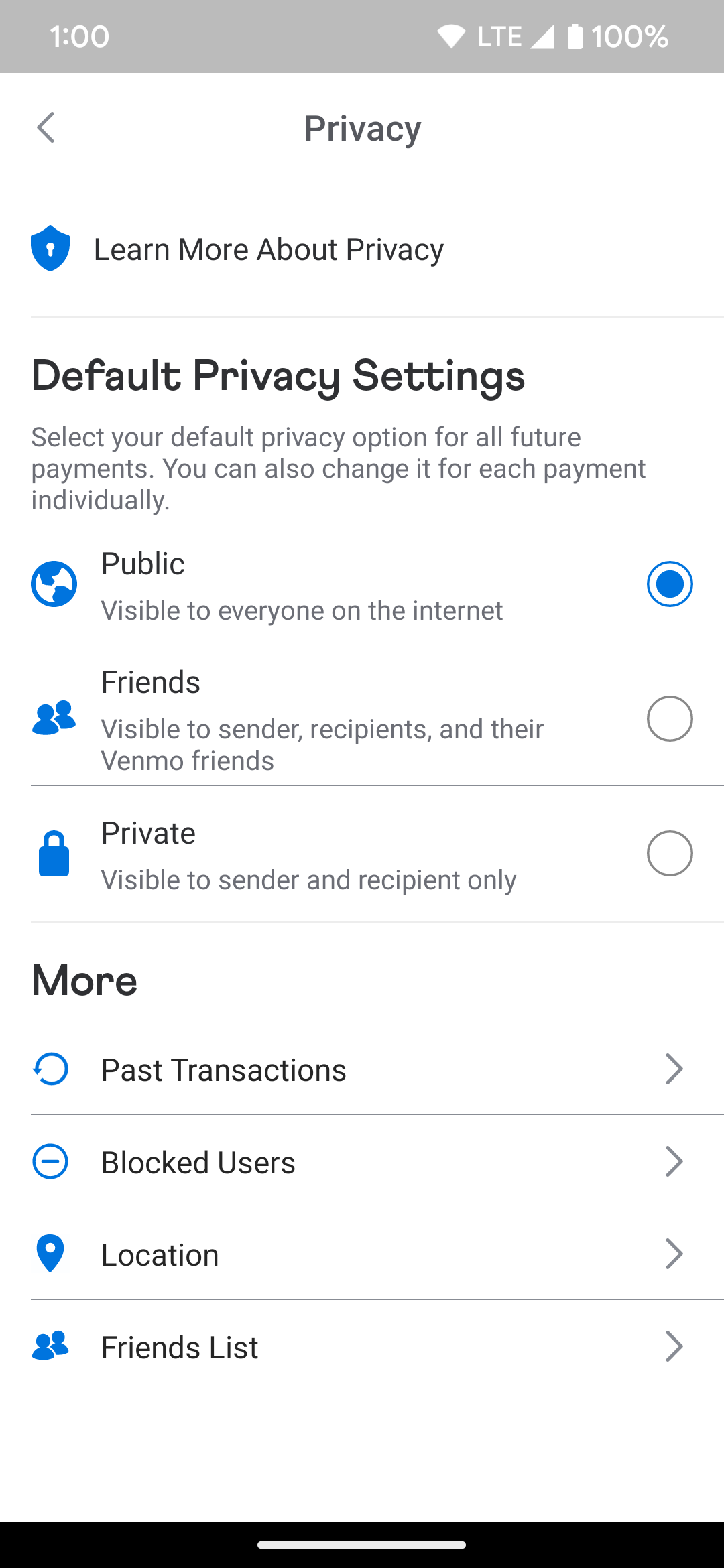Screenshot of a cell phone screen displaying privacy settings at 1 o’clock. The status bar shows icons for Wi-Fi, LTE, and a full 100% battery. Below this, an option to learn more about privacy is illustrated by a blue shield icon with a keyhole.

The "Default Privacy Settings" section allows users to choose a default privacy option for all future payments, but also to adjust privacy settings for individual transactions. The current setting is "Public," denoted by a globe icon and indicating that transactions are visible to everyone on the internet. 

Other available options include:
- "Friends," represented by an icon of two people, which makes transactions visible to the sender, recipients, and their Venmo friends (not selected).
- "Private," symbolized by a padlock icon, which restricts visibility to the sender and recipient only (also not selected).

Further settings options include "Past Transactions," "Blocked Users," "Location," and "Friends List," each accompanied by a right-pointing arrow indicating they can be accessed for more detailed settings.

A black rectangle with a small white horizontal line in the center appears at the bottom of the screen. The image is devoid of photographic elements, animals, or automobiles, and has a taller than wide aspect ratio.